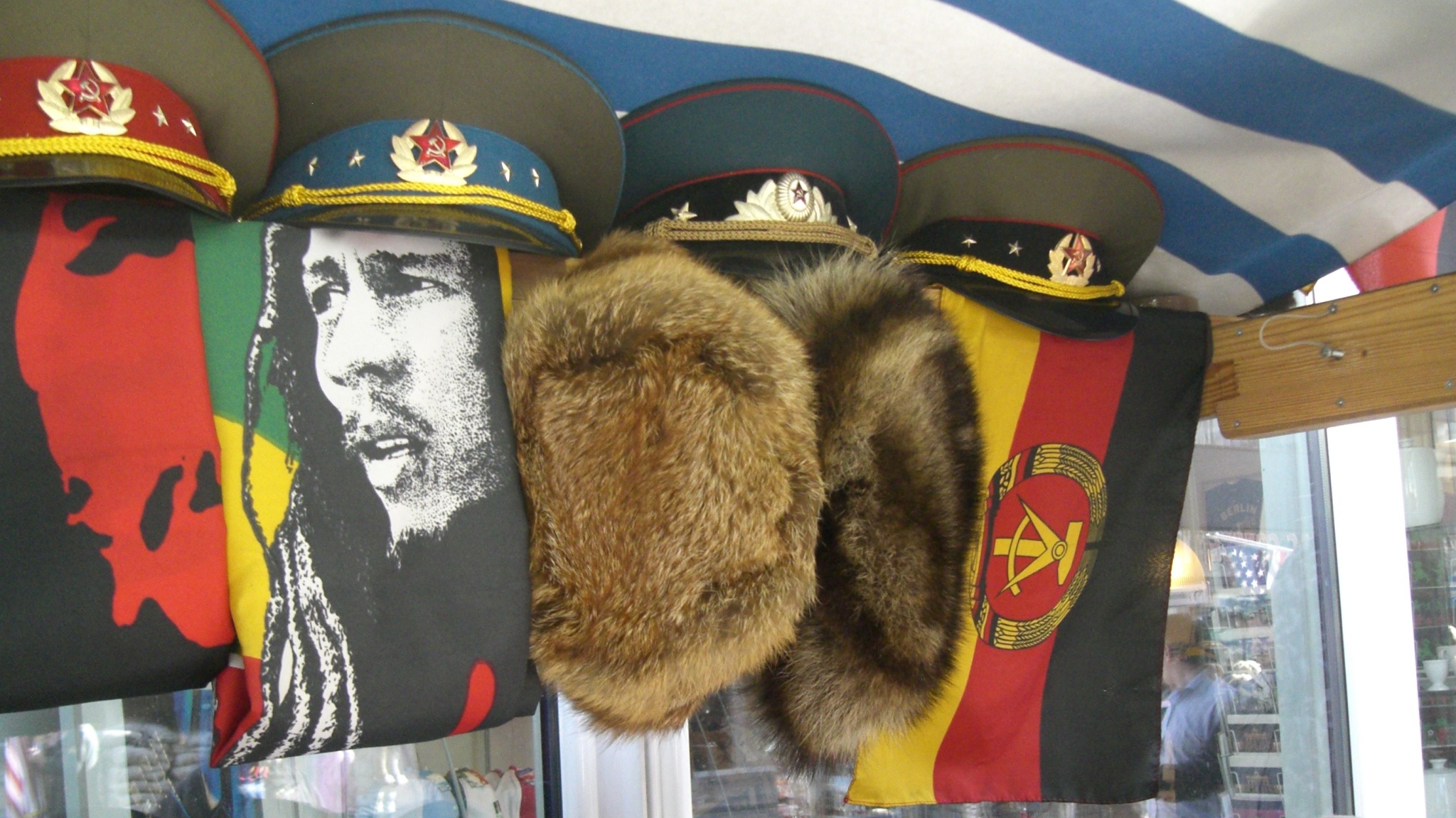The image depicts a display of military hats under a blue and white horizontally striped awning. Positioned on a ledge, the hats form a row starting from the upper left-hand corner of the picture. The first hat, partly cut off by the image edge, features an olive green top with a red band and two visible stars. Underneath, there's a piece of fabric, likely a tapestry, with a distinct red motif.

The second hat has an olive green top accented by a blue band adorned with four stars and an insignia in the center, featuring an open-ended wreath and a red star. Below this hat are two pieces of fur hanging, possibly fur caps.

The third hat, also olive green, displays a black band with a white emblem. Beneath it, there are two more fur pieces. 

Finally, the fourth hat has an olive green top with a black band and an insignia. Below it hangs a flag with vertical stripes in black, red, and gold, featuring a circle emblem in the center. To the right of the display, part of a glass door or wall is visible, along with a person standing and facing left. Above the door, a piece of wood extends from the right side of the image to the shelf holding the hats, completing the scene.